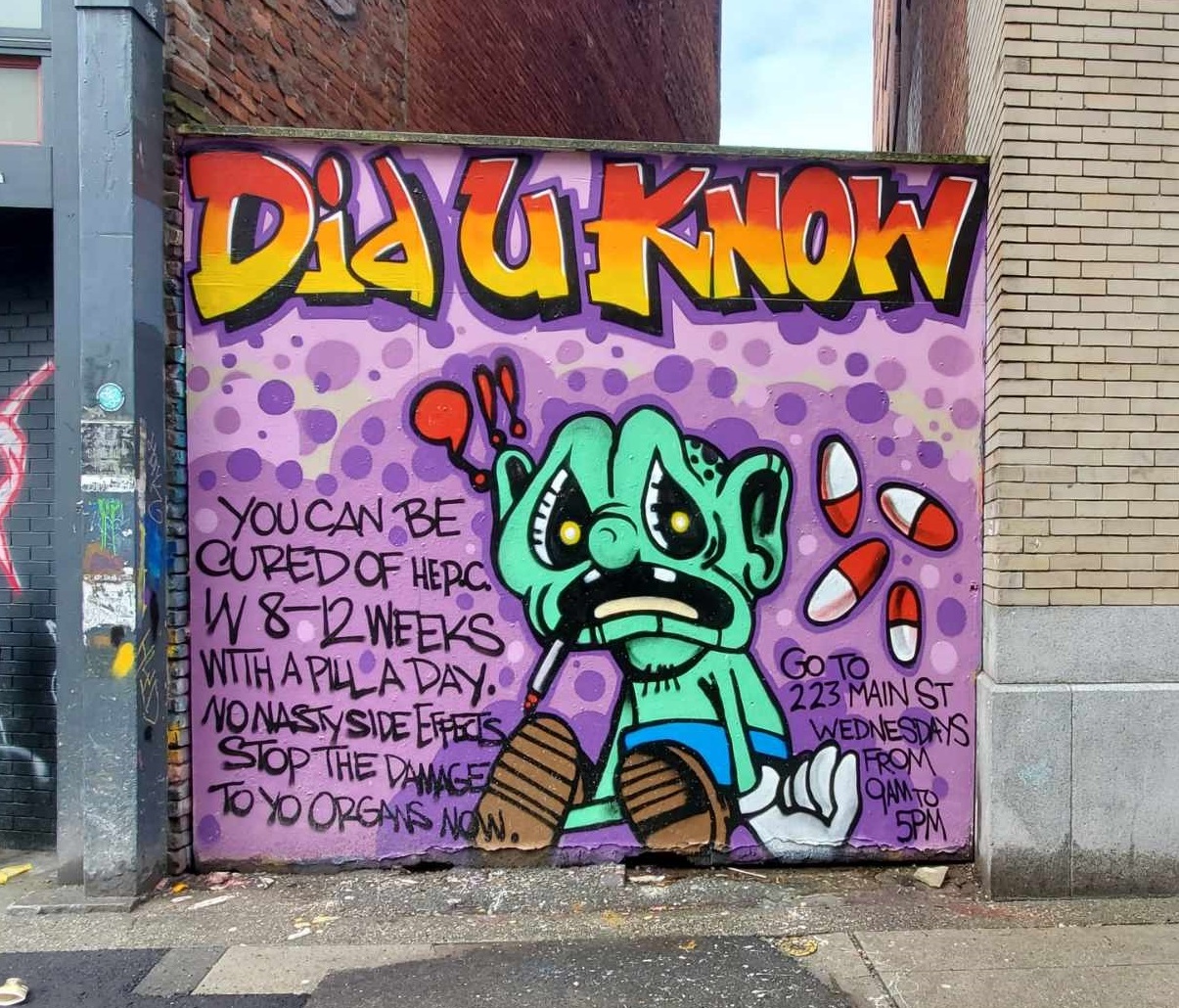The image depicts a large, eye-catching mural spanning a section of the wall between two buildings. On the left, the building has reddish-toned bricks, while the right side features an off-white to greyish stone structure. The mural prominently displays the text "Did You Know?" in a large, funky font that transitions from dark red at the top to yellow and orange at the bottom. Below this, there's a seated, green alien-like figure with big black eyes featuring yellow dots, and only two teeth. The alien looks perplexed, with a cigarette hanging from its mouth, donning blue shorts and brown shoes. Surrounding the alien are several large red and white pills. On the right side of the mural, black text reads, "You can be cured of Hep C within 8-12 weeks with a pill a day. No nasty side effects. Stop the damage to your organs now." Additional smaller text provides directions: "Go to 223 Main Street Wednesdays from 9am to 5pm." The mural's background transitions from a dark purple at the base with circular spots, to lighter shades of purple as it ascends towards the "Did You Know?" text at the top. This vivid and intricate mural aims to attract the attention of passers-by and provide important health information.